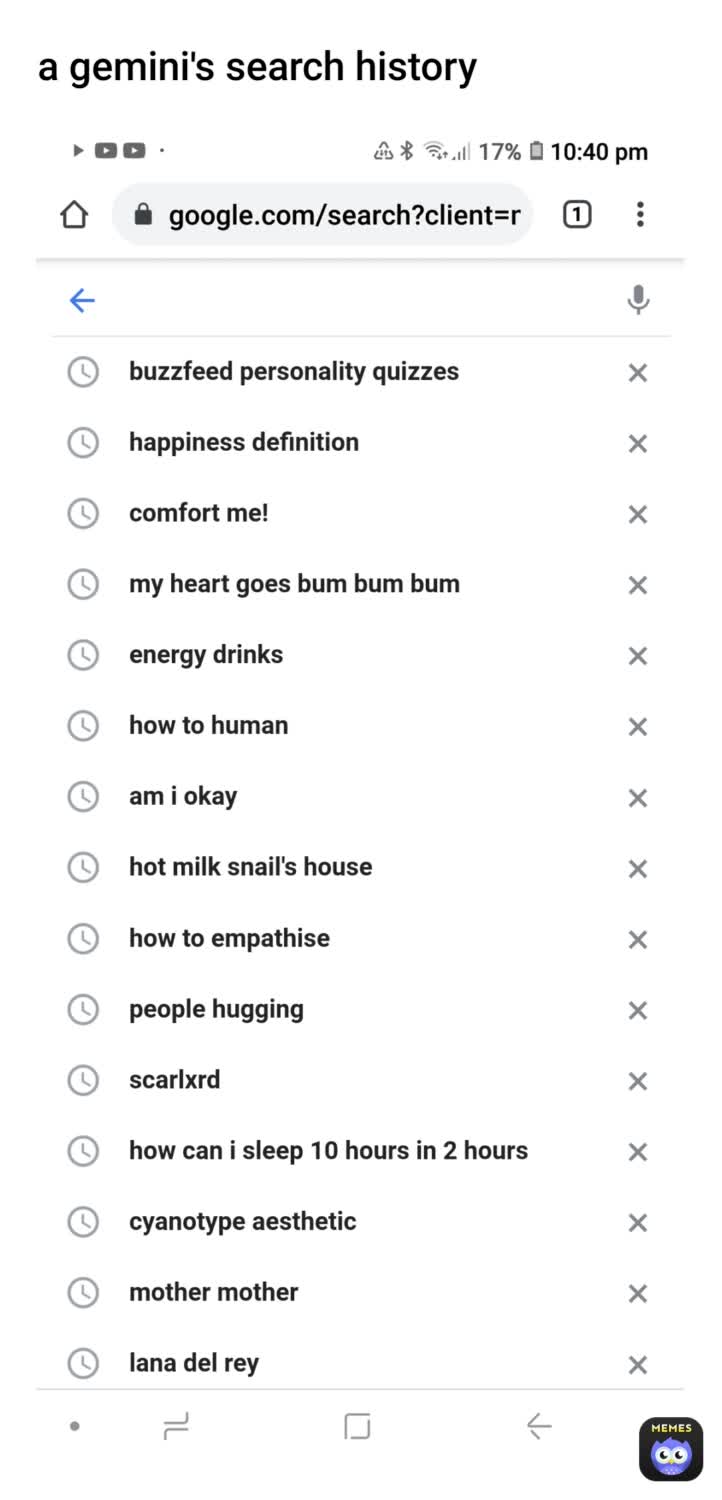Screenshot of a mobile phone search history with a white background and black text. The screenshot is slightly tinted with a light gray tone. At the top, it reads "Gemini search history," followed by status icons for Bluetooth, battery percentage (indicating 10:40 PM), and network signals. The list of search queries includes:

- BuzzFeed personality quizzes
- Happiness definition
- Comfort me
- My heart goes bum bum
- Energy drinks
- How to human
- Am I okay
- Hot Milk Snail’s House
- How to empathize
- People hugging
- Scarlxrd
- How can I sleep 10 hours in two hours
- Cyanotype aesthetic
- Mother Mother
- Lana Del Rey

Each entry is accompanied by a clock icon on one side and a close (X) icon on the other. In the lower corner is a blue owl icon with the word "memes."